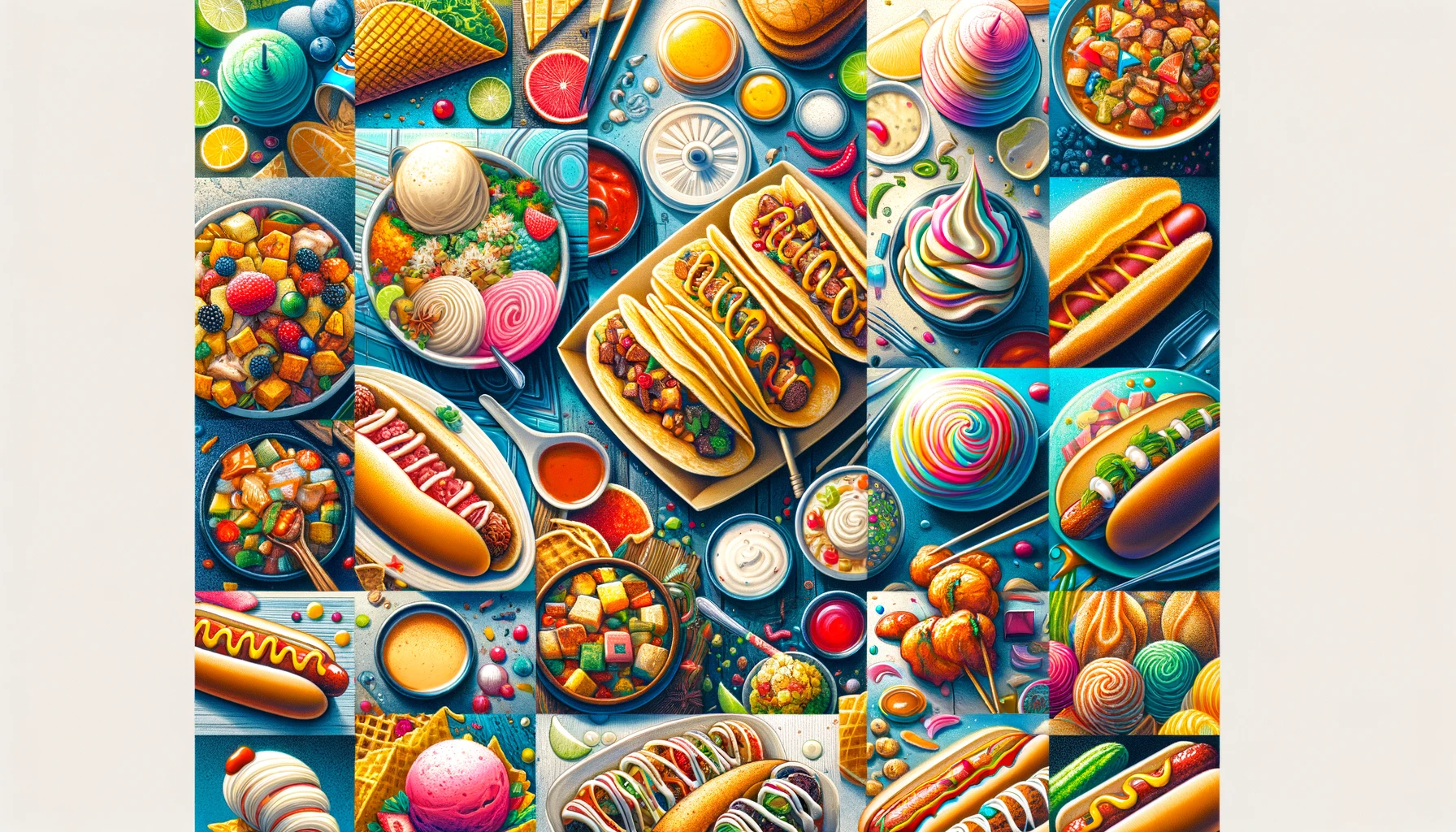The image showcases a vibrant and detailed digital illustration of assorted junk foods, characterized by bold and bright rainbow colors. The scene is composed in a landscape orientation, set against a light gray backdrop. The main composition features a collage of smaller, square illustrations arranged in a grid, each depicting a variety of snack items.

Prominently, the image includes six hot dogs, three tacos on a plate centered in the middle, and a cereal bowl with fruits. Scattered around, you can find soft swirl ice cream cones, scoops of ice cream accompanied by colorful round cookies, and waffle ice cream topped with muffins. There are also colorful soups filled with cubes and beans, fruit salads, and regular salads, alongside dips and cupcakes.

The cohesive aqua-toned background enhances the lively presentation of the foods, with the dominant colors being brown and blue. Each section of the image is meticulously detailed, making the junk foods appear both delightful and exaggerated in their cartoonish style. The overall effect is a mesmerizing array of street foods and desserts, vividly illustrating a feast for the eyes.